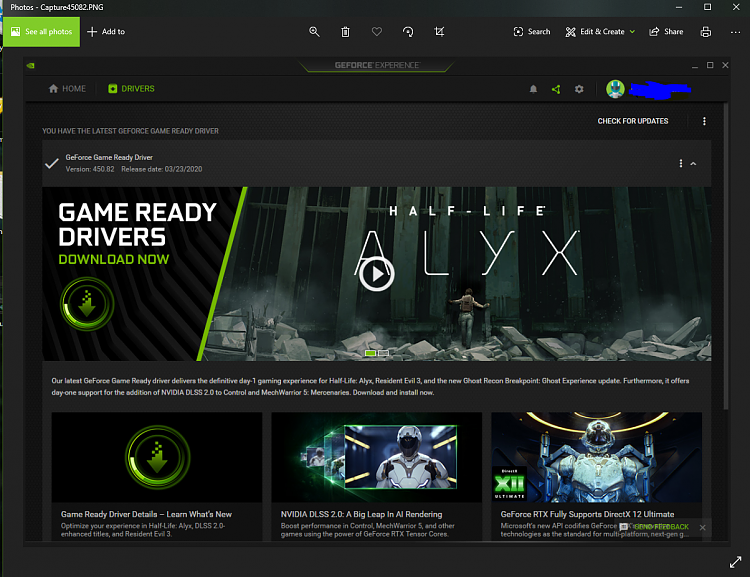This is a detailed screenshot from the GeForce Experience application, showcasing an update feature for GeForce drivers. The background is gray, and in the upper left corner, you can see the file name "photos-capture-550A2.PNG" displayed. Below this, there is a yellow rectangle with white text that reads "See All Photos" and a white plus sign indicating "Add To," forming an overlay of how the screenshot was taken.

At the center top, the GeForce Experience logo is prominently displayed. Beneath the logo, there are two navigation buttons labeled "Home" and "Drivers," with the "Drivers" button currently selected.

In the upper right corner, there's a user profile icon depicted as a cartoon character wearing a motorcycle helmet. Below the profile picture, light gray text reads, "You have the latest GeForce Game Ready Driver."

Further down, there's a lighter gray rectangle providing specific driver information: "GeForce Game Ready Driver version 450.82, Release Date: 01/23/2020."

At the bottom of the screenshot, a banner with a call to action states "Game Ready Drivers Download Now," featuring a video thumbnail of "Half-Life: Alyx."